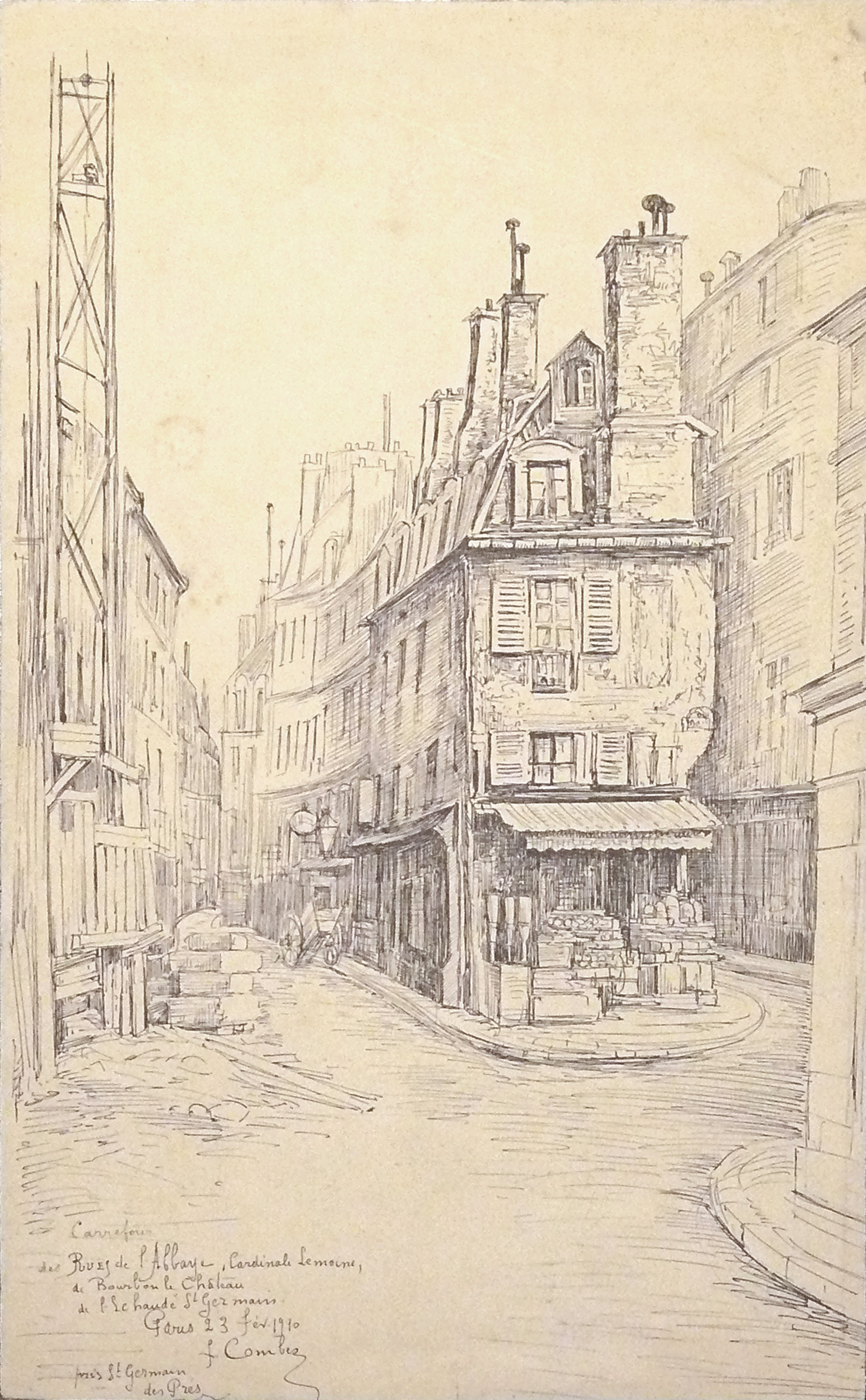The image is a detailed black and white sketch, in pen and ink, depicting a European city street scene. The perspective is from a street that forks in two directions, bordered by tall, older buildings that appear slightly tarnished from age. Dominating the scene is a central row of interconnected buildings, with a distinct storefront at the forefront displaying consumer products. The left side of the image features a prominent tall building, with boxes stacked near its lower section. To the right, another imposing structure showcases shutters and a market with a white awning below. The entire scene is shaded to create a stark contrast between the black and white elements. Chimneys rise from the rooftops, stretching into the pale white sky typical of a light whitewash sketch. At the bottom left corner of the image, a cursive text provides some information, though it is hard to read, indicating perhaps the name of the author or illustrator. The image is devoid of human figures and conveys a serene, slightly hazy ambiance of an old city landscape.